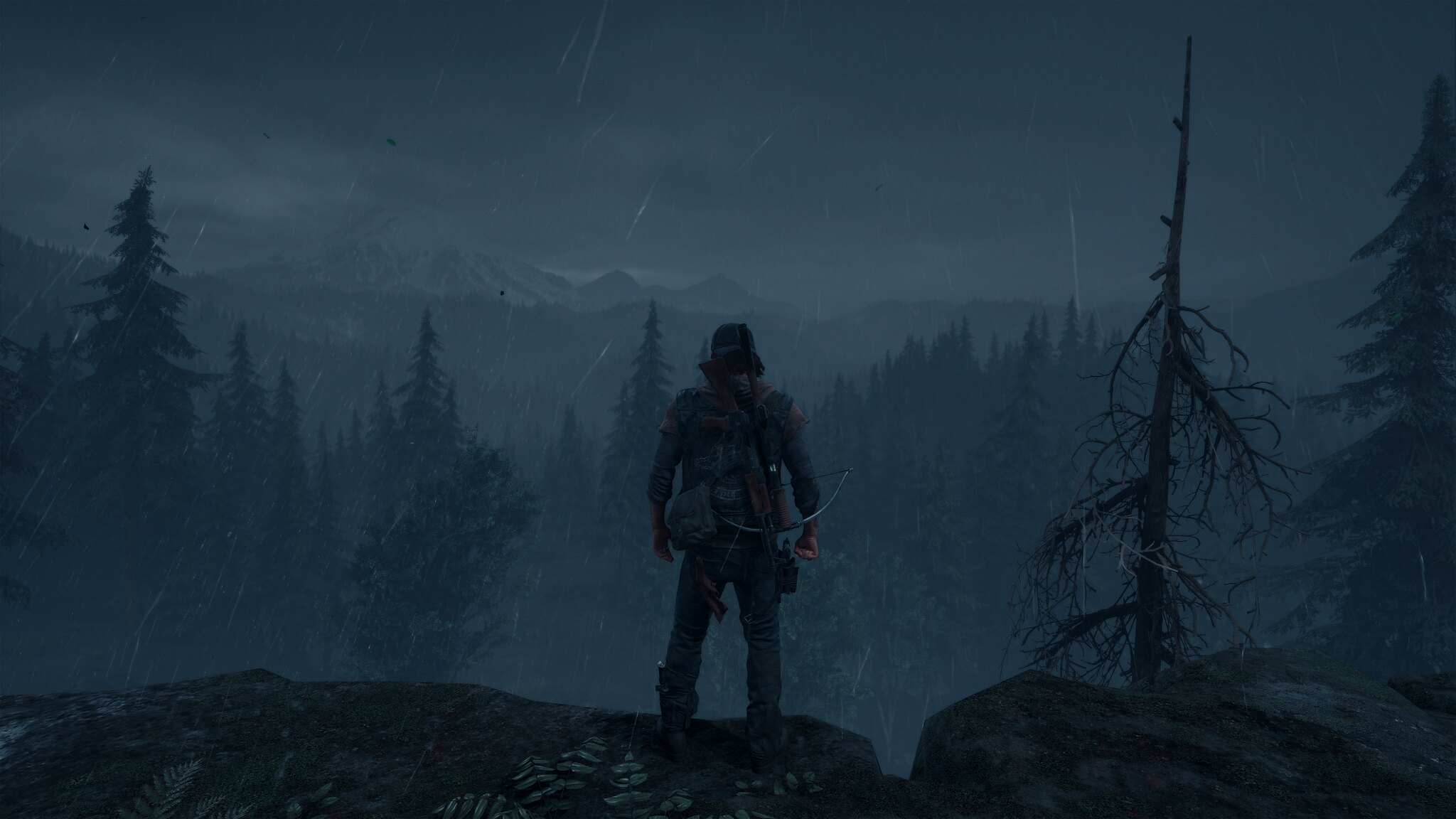The image appears to be a highly realistic and detailed computer-animated screenshot, possibly from a game, depicting a white male character standing on the edge of a rocky cliff. He is dressed in green denim pants, a brown and gray shirt, a blue denim jacket, and a gray trucker hat worn backward. The character has a pack on his side and carries a powerful, bow-like gun on his back. The setting is a mountainous landscape shrouded in dark gray, cloudy, and hazy skies, with hints of rain indicated by white streaks. A bare tree, stripped of leaves, stands to his right, contrasting with the lush green-leaved trees in the distance. The horizon features layers of treetops and a snow-capped mountain peak, creating a dramatic and expansive view. The character's pose suggests he is surveying the scenery, adding a dynamic sense of adventure and exploration to the scene.